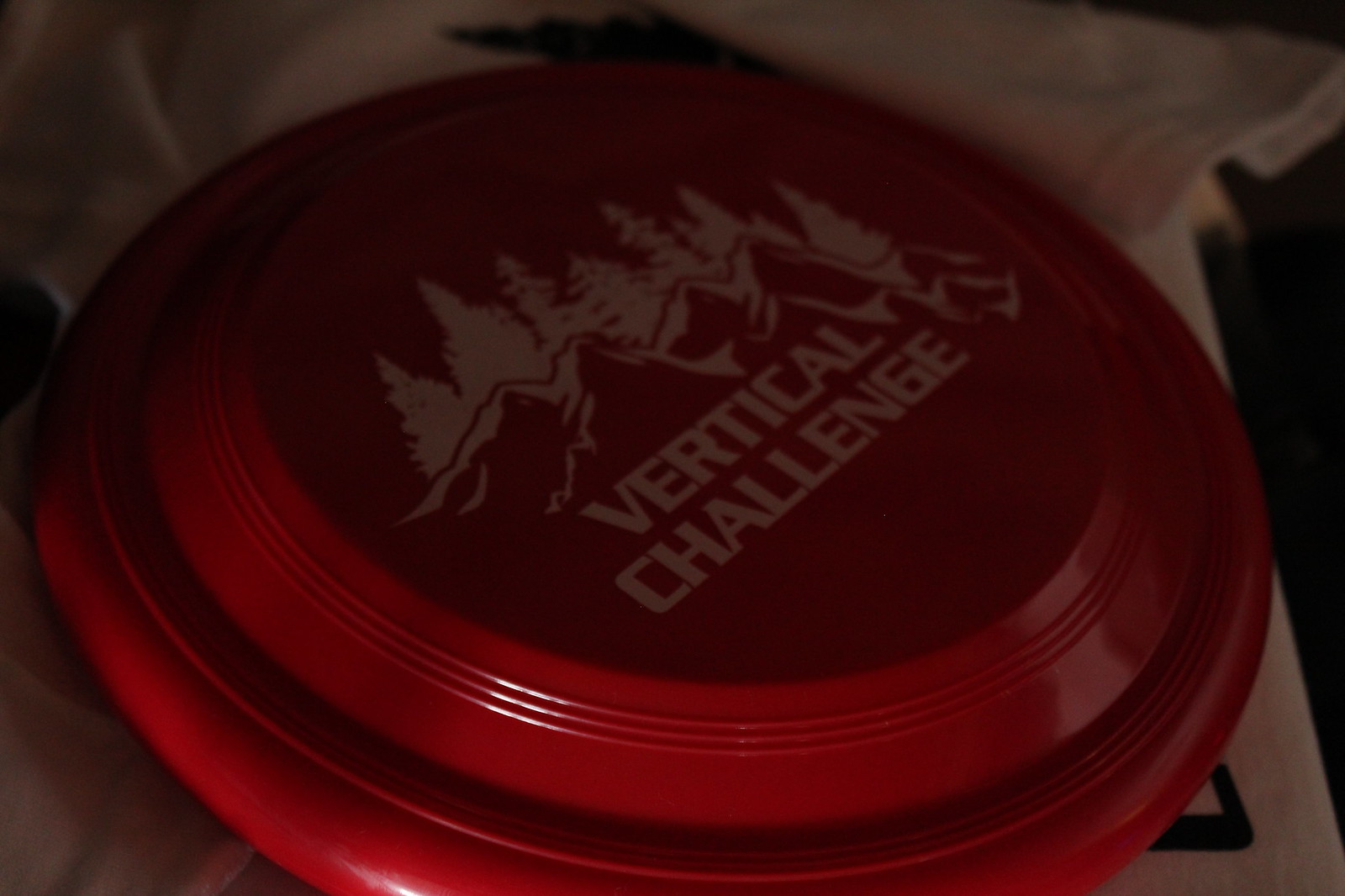This photograph captures a dark, dimly lit scene with minimal light, likely taken in a room with a single light source coming from the lower left. At the center of the image is a prominent red frisbee or flying disc, which takes up the majority of the frame. This frisbee, which appears to be slightly higher in the middle than a typical frisbee, features an intricate design. The design consists of a mountain pattern with five distinct mountains and several smaller rock formations, all set against a backdrop of tall white trees. Below this picturesque scene, the words "VERTICAL CHALLENGE" are emblazoned in white capital letters. The frisbee is positioned atop some sort of booklet and partially drapes over a white piece of cloth, possibly a t-shirt. The overall impression of the photograph is one of subdued lighting with the focus squarely on the detailed and uncommon red frisbee.